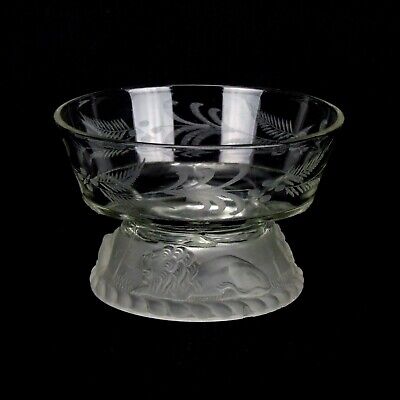The image depicts a clear glass bowl set against a completely black background. The bowl is divided into two sections: the upper transparent portion adorned with shiny, reflective patterns of wheat and leaves, and the base, which is frosted glass with a knotted rope design. At the front of the base, there's an intricate relief of a lion positioned with its head to the left, its hind parts to the right, and its tail curling upwards around its body. The base appears heavy and slopes inward to support the clear, decorative bowl above it. Two light sources reflected in the glass lend a glistening quality to the whole piece.